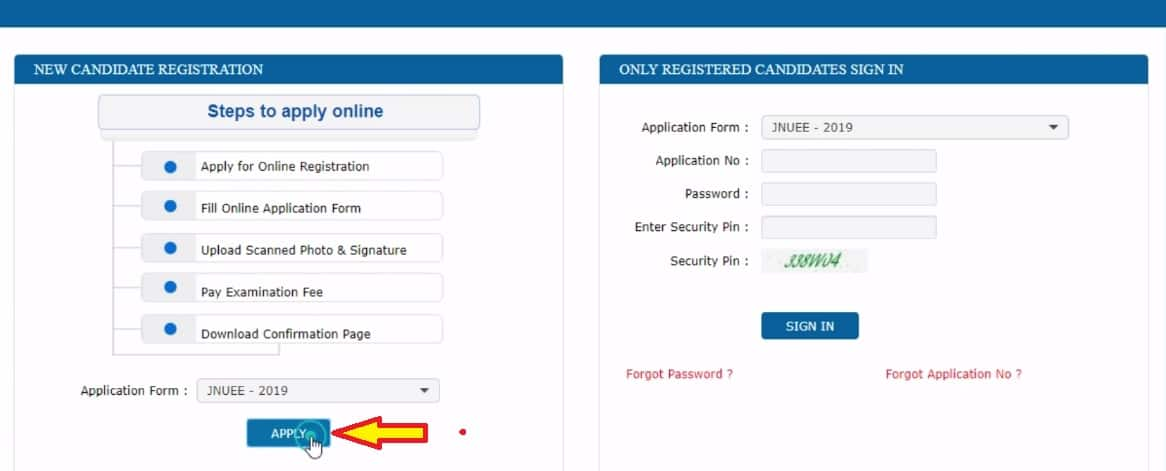The webpage features a clean and organized layout, starting with a blank blue banner at the top. Directly below the banner, the page is divided into two sections for user interaction. 

On the left side, the section is dedicated to new candidate registration. It begins with a blue banner labeled "New Candidate Registration" in white text. Below this banner is a white section titled "Steps to Apply Online" in blue lettering. Here, five buttons are vertically listed, each guiding the user through necessary steps: "Apply for Online Registration," "Fill Online Application Form," "Upload Scanned Photo and Signature," "Pay Examination Fee," and "Download Confirmation Page." Beneath these options is a drop-down menu displaying "JNUEE-2019" as the selectable application form. An accompanying blue "Apply" button shows a finger pressing it, highlighted by a yellow arrow outlined in red to its right.

On the right side of the page, a blue-bordered box is labeled "Only Registered Candidates Sign In" in white text. This area offers fields for user credentials and identification: "Application Form" (pre-set to "JNUEE-2019" as a drop-down option), "Application Number," "Password," and two fields for security verification— "Enter Security PIN" and a displayed "Security PIN" with the value "338W04." A prominent blue "Sign In" button with white text is positioned beneath these fields. Below the "Sign In" button, two red links offer assistance, labeled "Forgot Password?" and "Forgot Application Number?" respectively.

The structured layout provides clear, step-by-step instructions for new registrations on the left, while facilitating easy access for returning users to sign in on the right.